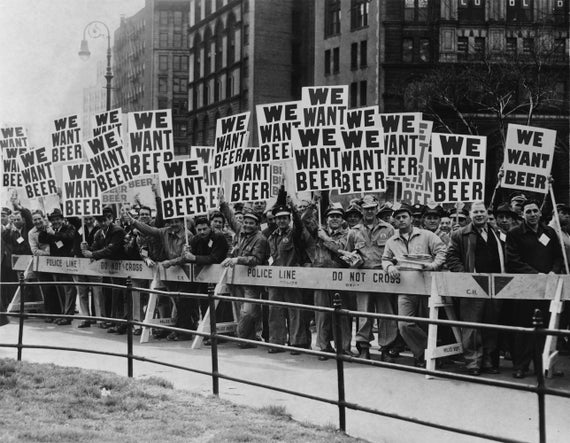This black-and-white photograph, likely taken during the Prohibition era, captures a large outdoor protest in a city. The demonstrators, predominantly men, are positioned behind a wooden police barrier labeled "Police Line Do Not Cross." The crowd comprises a mix of everyday working-class individuals, some clad in work jumpsuits, military hats, business suits, or sweaters, emphasizing their diverse backgrounds. Each protester holds a sign in large font reading "We Want Beer," expressing their unified demand. The backdrop features several tall buildings ranging from six to eight stories high, interspersed with tall street lamps. The scene appears to be set on a cloudy day, further enhancing the historical atmosphere of the image.